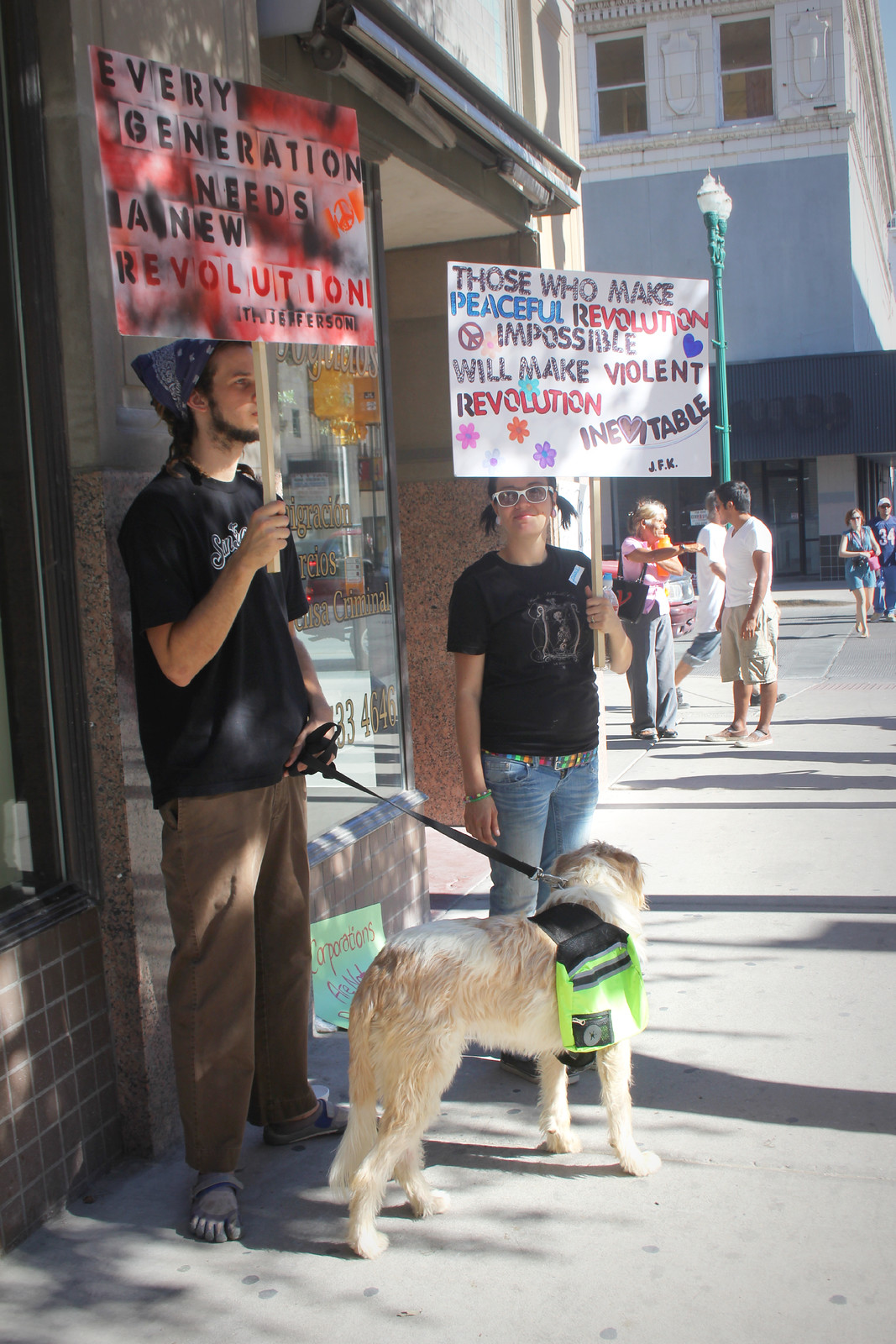In this photograph, two individuals are standing on a sidewalk holding banners. The person on the left holds a banner that reads, "Every generation needs a new revolution," while the person on the right displays a banner with the message, "Those who make peaceful revolution impossible will make a violent revolution inevitable." The individual on the right is also holding a leash attached to a dog, which stands obediently beside them. Both individuals are dressed in black t-shirts. In the background, a few other people can be seen either standing or walking. To the left side of the sidewalk, several buildings are visible, providing an urban backdrop to the scene.